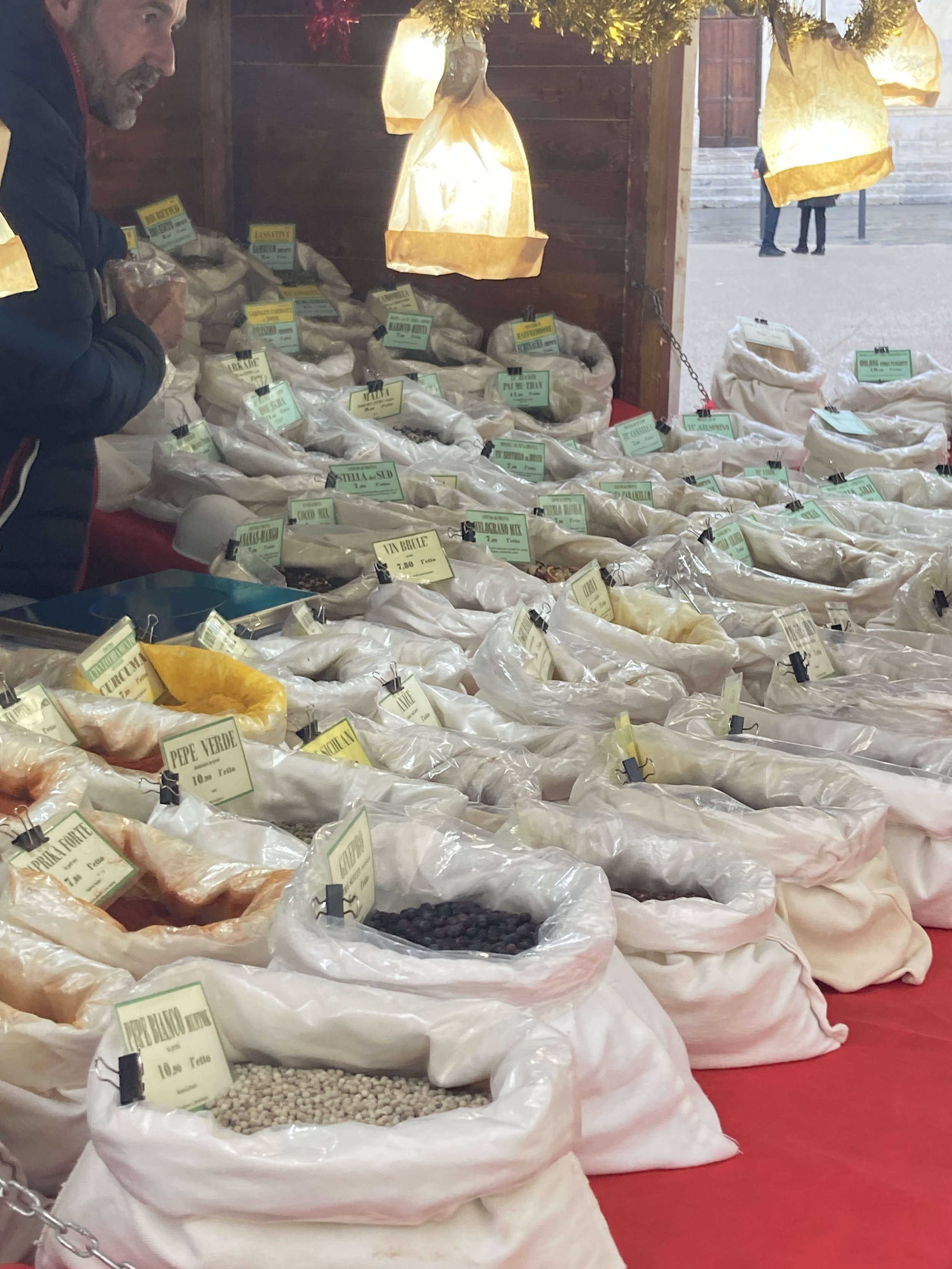In this bustling open market scene, a Caucasian gentleman with a slight beard stands behind a table covered with a red cloth. He is dressed in a dark blue jacket and appears on the upper left side of the photo. The table is laden with around 30 to 40 white sacks, each neatly curled down at the top and tagged with labels. These sacks contain a variety of items, including beans, seeds, and spices. The visible contents include black beans, a reddish-colored powder, and possibly gray beans. Among the labels, "Pepe Verde" and "Pepe Blanco" can be discerned, hinting at the variety of products offered. Above the table, bags hang like lanterns with lights inside, adding a unique touch to the vibrant market atmosphere. In the background, a doorway leads out to the street, where the feet of passersby can be seen. The gentleman, whose expression is obscured by his slight beard, has a metal object or briefcase in front of him, suggesting a well-prepared merchant engaged in his trade.